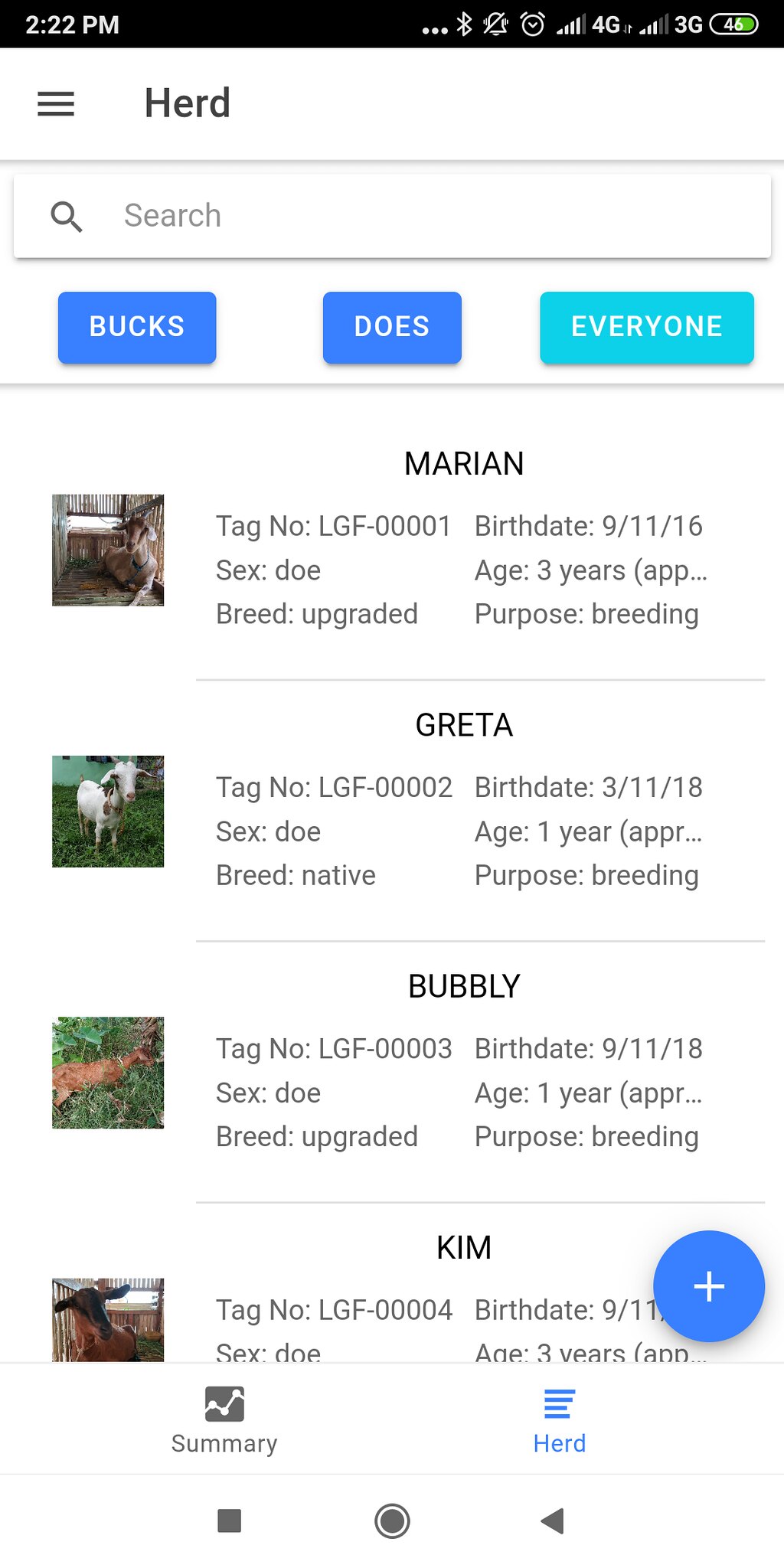The image is a detailed screenshot of a phone displaying an app or website called "Herd." The timestamp on the phone reads 2:22 p.m., and the device shows full bars of connectivity with both 4G and 3G networks, and a battery level at 46%. The status bar at the top displays several icons, including Bluetooth, silent mode, and an alarm clock.

Below the status bar, the screen features the name of the app "Herd" in a black background. It includes a search bar and three blue buttons labeled "Box," "Us," and "Everyone," with the "Everyone" button highlighted.

The main content on the screen shows a list of goats with details for each. On the left are images of the animals, and on the right are their individual information. The listed goats are:
- Marion: Tag number LGF00001, Sex: doe, Breed: upgraded, Birth Date: 09/11/2016, Age: approximately 3 years, Purpose: breeding.
- Greta: Tag number LGF00002, Sex: doe, Breed: native, Birth Date: 03/11/2018, Age: approximately 1 year, Purpose: breeding.
- Bubbly: Tag number LGF00003, Sex: doe, Breed: upgraded, Birth Date: 09/11/2018, Age: approximately 1 year, Purpose: breeding.
- Kim: Tag number LGF00004, Sex: doe, Birth Date: partially obscured, Age: approximately 3 years, Purpose details partially obscured.

The bottom of the screen shows navigational icons, including a summary button on the left, the name "Herd" with four blue lines above it on the right, and system navigation buttons such as back, home, and recent apps.